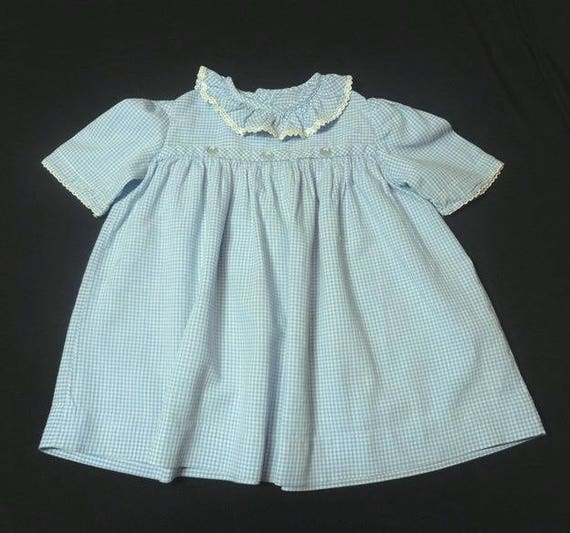This photograph showcases a vintage, pale blue infant gown, likely dating from the 1980s, laid out on a dark grey to black background. The gown features a delicate, lace-trimmed collar and short sleeves edged with lace. The fabric has a subtle white dotting pattern, contributing to its slightly antique look. Decorative non-functional buttons adorn the chest area, adding to the dress's ornate charm. Despite its elegant design, the material appears a bit dingy, suggesting it could be a collector's item. The dress, centered in the image, evokes the style of meticulously crafted children's apparel from past decades, potentially spotted in online listings.